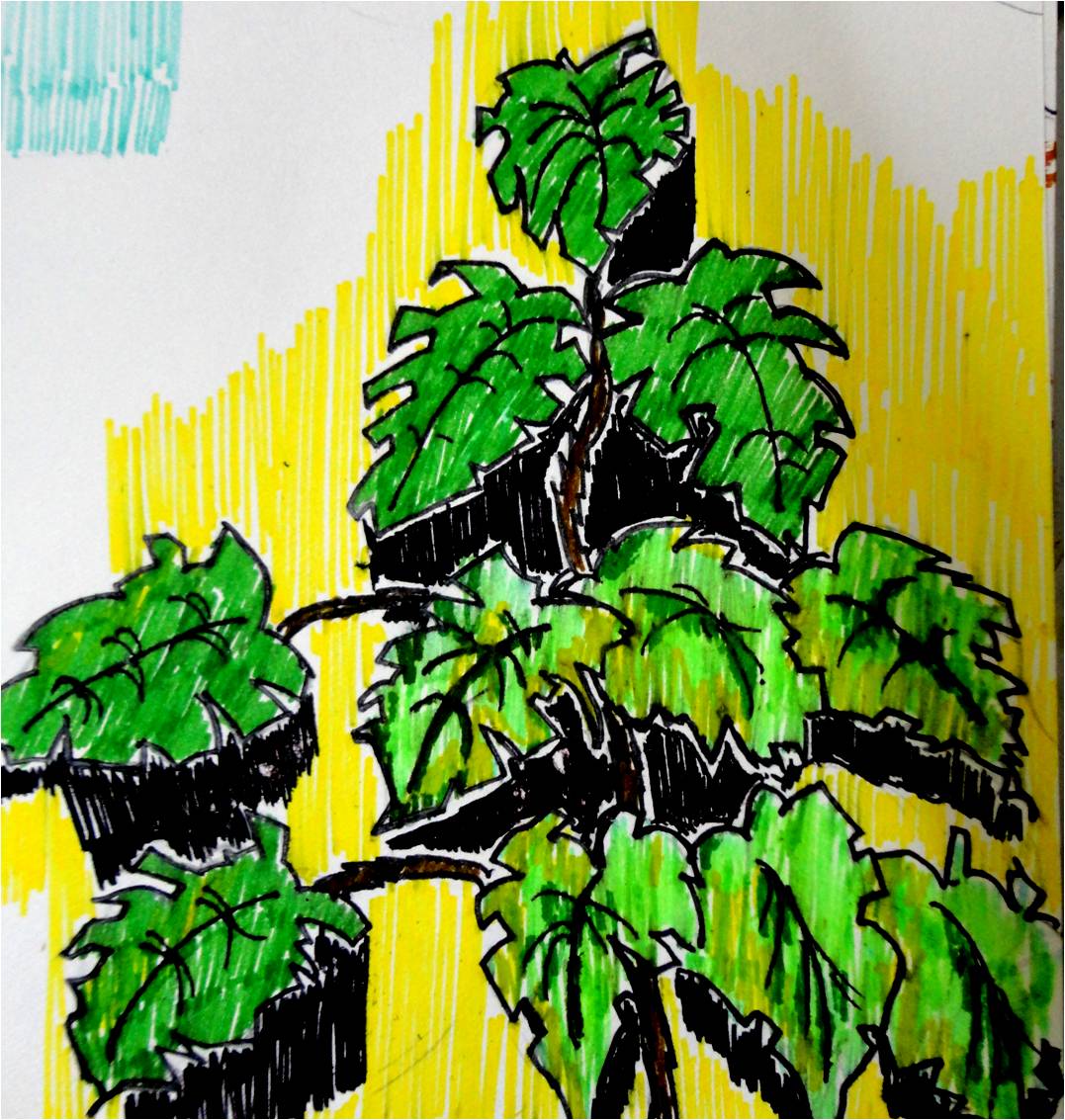The image is a detailed color marker drawing of a bushy plant on white paper. The plant features approximately 10 jagged-edged, medium green leaves, shaded with light green and yellow hues towards the bottom. Each leaf is outlined and veined in black marker, contributing to a vivid, detailed appearance. The stems, primarily brown, are visible toward the top part of the plant, and the image is enhanced with black shading below the leaves for added depth. The plant lacks a visible pot or main stem, extending off the bottom right-hand part of the image. The background is marked with vertical yellow stripes created by a magic marker or pen, save for the upper left corner, which contains a faint blue square, possibly symbolizing the sky.